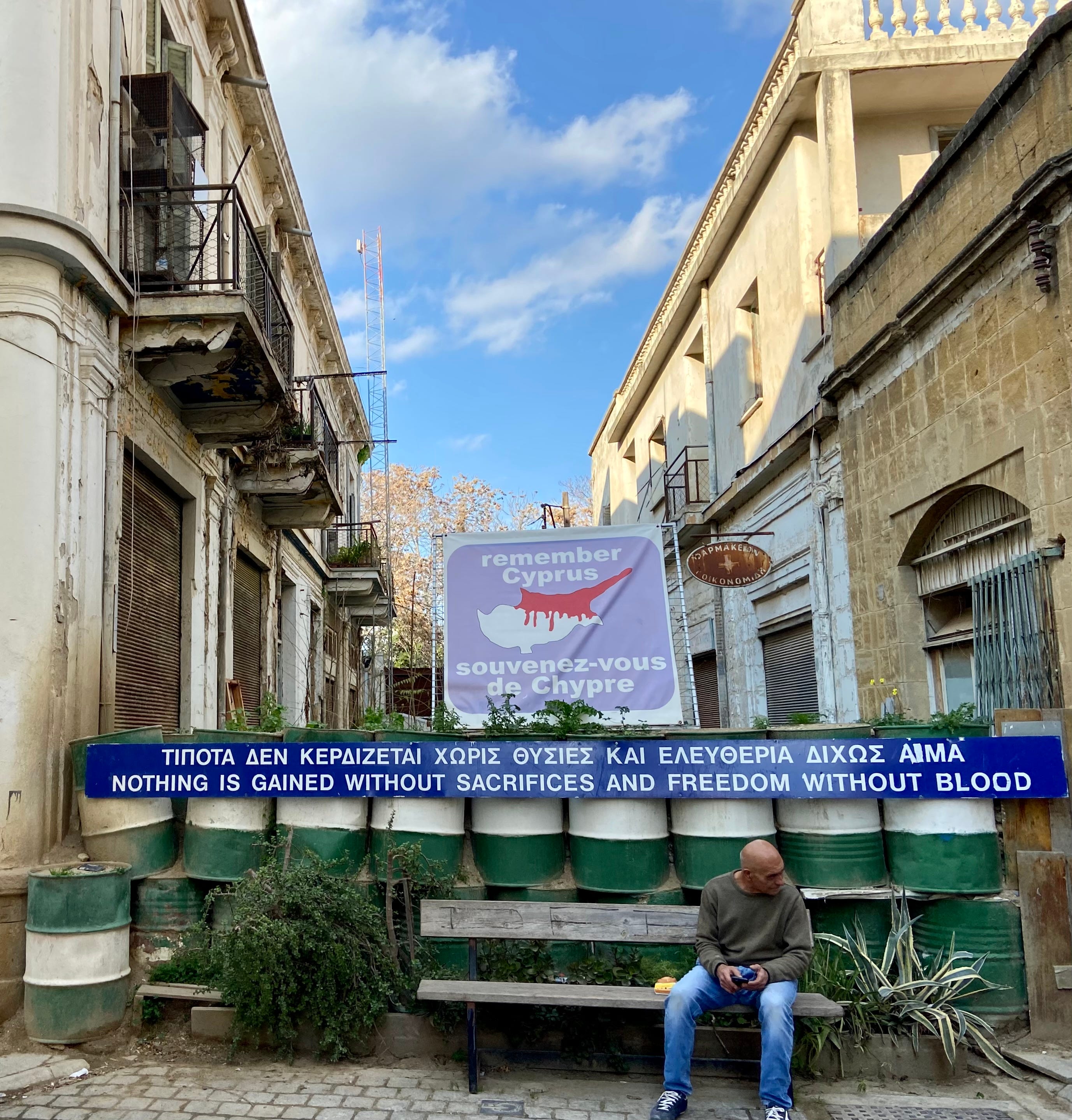The outdoor daytime color photograph captures a scene at street level, focusing on an alleyway framed by two two-story buildings—one displaying classical ornate stonework and balconies on the left, and a more modern structure with a series of windows on the right. In the foreground, a man dressed in jeans and a green shirt sits on a park bench, looking to his left. The cobblestone street beneath the bench and the plants behind it add to the everyday urban ambiance. Directly behind him is a row of eight or nine green and white 55-gallon drums, aligned neatly in a row. Stretching across the front of these drums is a blue banner, which is inscribed with text in both Russian and English. The English text delivers a powerful message: "Nothing is gained without sacrifices and freedom without blood." Above this, another blue banner attached to a frame reads, "Remember Cyprus," in white lettering. The sky visible between the buildings is a clear blue with scattered white clouds, completing the scene. This combination of architectural details and evocative signage suggests a setting rich in historical and political context.